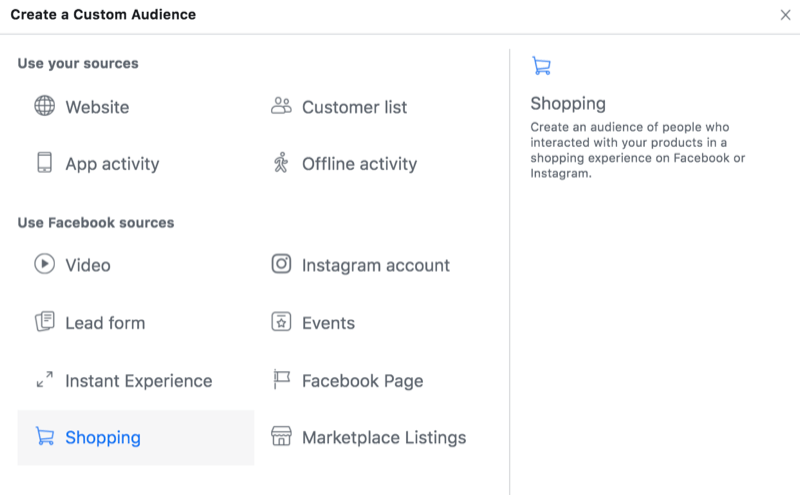This image depicts a clean, white-background e-commerce website, possibly showing a pop-up or overlay screen. In the upper left corner, black text reads "Create a Custom Audience." Below that is a large square section with several links.

The first section within the square is titled "Use Your Sources" and includes the following links:
- Website
- Web Activity
- Customer List
- Offline Activity

Immediately beneath this is a second section titled "Use Facebook Sources," featuring these links:
- Video
- Lead Form
- Instant Experience
- Shopping
- Instagram Account
- Events
- Facebook Page
- Marketplace Listings

To the right of this square section is a tall rectangular section. It has a blue shopping cart icon at the top left, followed by the word "Shopping." Below the icon, the text describes, "Create an audience of people who interacted with your products in a shopping experience on Facebook or Instagram."